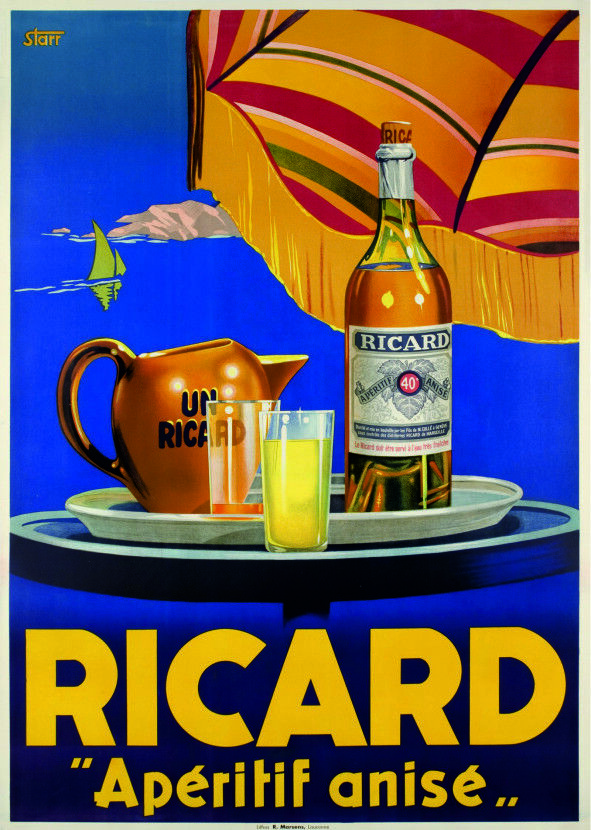The image appears to be an animated or computer-generated etching, showcasing a promotional scene for an alcoholic beverage. On the right side of the composition, there is a distinctive bottle with a green-colored glass containing an orange liquid. The bottle is sealed with a brown cork and has a gray wrapping just below the cork. Prominently displayed on the bottle is a white label that reads "Ricard" at the top, with a red circle in the center containing the number 40.

In the center of the tray, there are two clear crystal glasses. One of these glasses is filled with a yellow liquid, while the other remains empty. Positioned behind the glasses is a picture in a gold frame with black letters that spell out "Un Ricard."

The entire setup is arranged on a black circular table. Below the image, in light orange lettering, it reads "Ricard". Further text below states "A-P-E-R-I-T-I-F E-N-I-S-E."

The background is designed to resemble a marine scene with a green sailboat navigating through what appears to be dark blue ocean waters, enhancing the thematic emphasis on the Ricard aperitif in an idyllic setting.